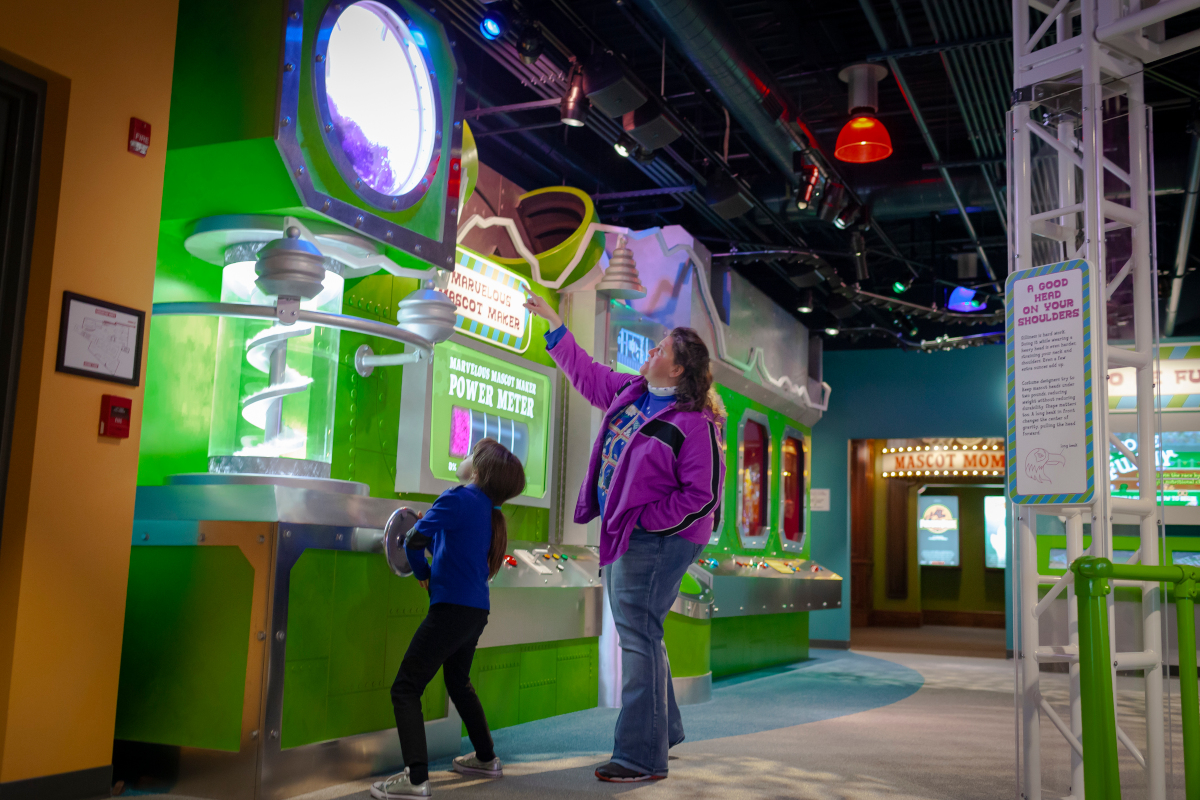The photograph depicts a lively scene in an arcade setting, possibly also a science museum, featuring a woman in a light blue coat and blue jeans, accompanied by a young girl in black pants, a light blue shirt, and Converse sneakers. Dominating the image is a striking green machine, which the child is interacting with, steering a wheel to control purple goo visible through a circular glass window at the top. Below the goo chamber, a spiral tube runs through a large glass cylinder. The machine is labeled "power meter" and "marvelous mascot maker." The background is detailed with an orange wall on the left, featuring a red fire alarm and a white picture in a black frame, while the right side includes various other arcade games and a green column. A prominently visible sign reads "a good head on your shoulders," framed by a light blue and yellow border with an image of a bird. The scene is vibrant, with lots of engaging elements that capture the playful and educational atmosphere.